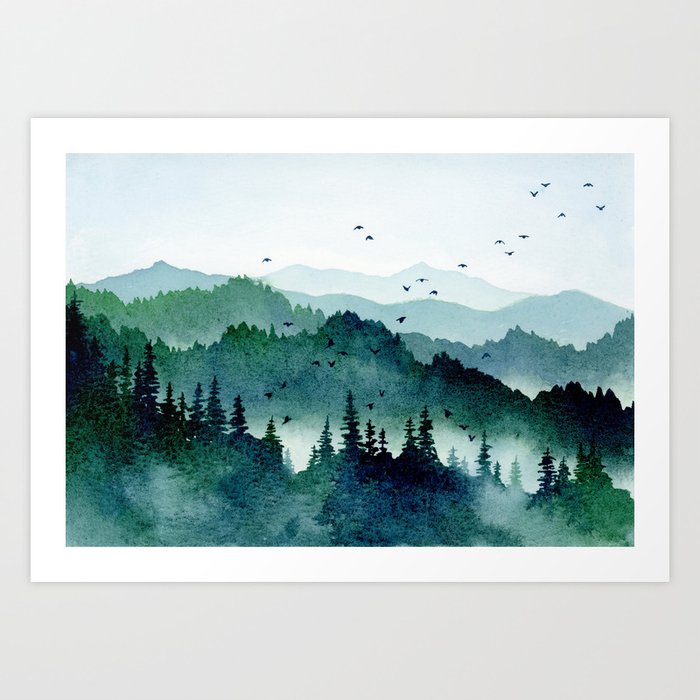This watercolor painting captures a serene and scenic landscape adorned with delicate layers of color and detail. The image is square with the painting centered inside of a white-bordered rectangle against a gray background. The main illustration portrays a tranquil scene moving from a dark, silhouetted foreground to a misty, almost ethereal background.

In the immediate foreground, a dense row of blackish trees interspersed with hints of dark green and blue sets a profound contrast. A subtle white smokiness imbues a sense of mist or dawn light, enhancing the scene's tranquil beauty. Moving further into the mid-ground, these trees begin to lose their sharpness and detail, blending into forms that resemble a mountain range. The gradient continues as the line of trees lightens, transitioning to shades of light blue and green. This gradient effect lightens progressively until the final range appears almost white, evoking a distant mountain peak merging with the sky.

The sky itself is a gentle, light blue, dotted with approximately twenty small bird silhouettes flying in various directions across the canvas. These elements, combined with the repeating blues and greens, create a harmonious and peaceful scene. The artistic touch gives the painting a dreamy quality, making it a compelling blend of realism and abstraction.